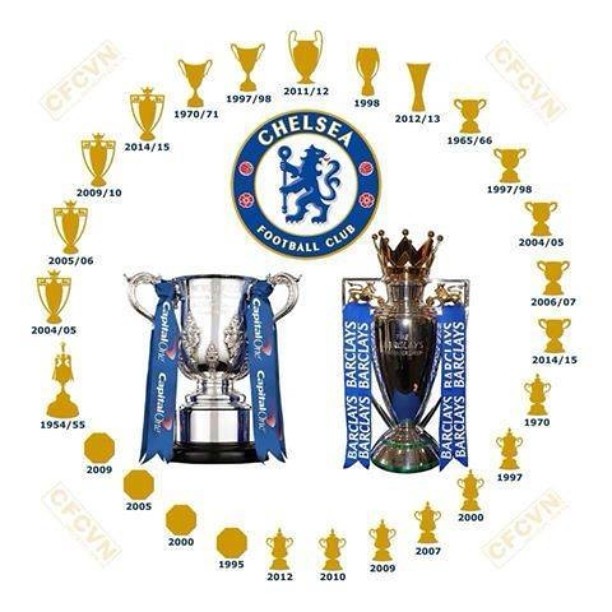The image showcases the Chelsea Football Club's emblem and a display of trophies commemorating their winning years, with dates ranging from 1965 to 2012. At the center, the Chelsea Football Club logo, featuring a dragon-like figure within a sky-blue circle, dominates the scene. Encircling the logo are outlines of various gold medals and trophies, each marking significant championship years like 2011, 1999, and 1998.

Positioned to the left and right below the emblem are two prominent trophies. On the left, there's a grand silver trophy with an expansive open cup, dual handles, and a substantial black base, adorned with blue Capital One ribbons. On the right stands a more brass-colored trophy, its top resembling a crown. This trophy features ornate handles, one resembling a lion and the other a bull, with blue Barclays ribbons trailing down. The trophies and the logo are centrally placed within the image, highlighting the club's celebrated victories over the years. The overall color scheme is dominated by shades of blue, white, and gold, reflecting Chelsea's iconic colors and their legacy of excellence.